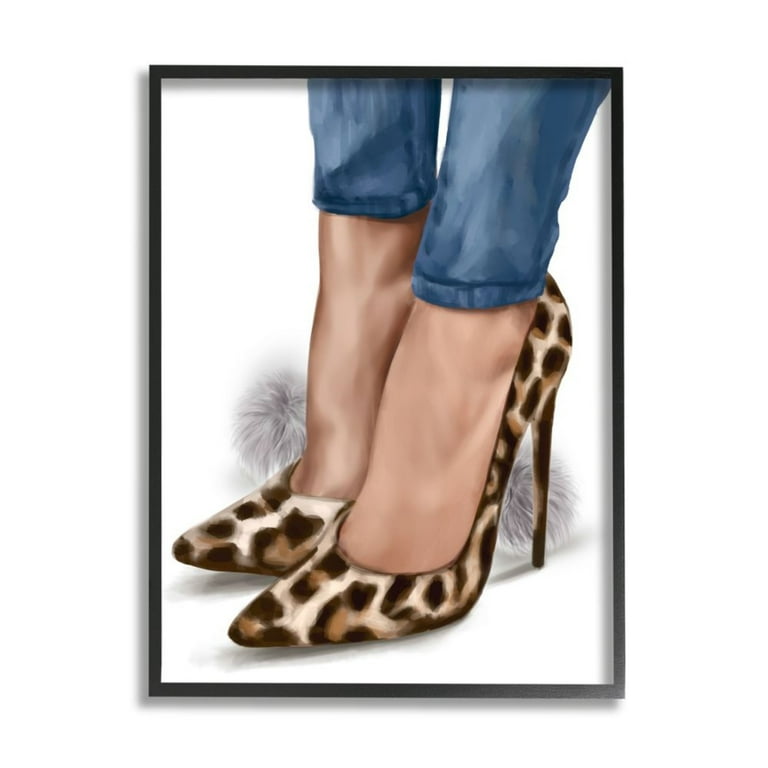This is a detailed, rectangular portrait measuring approximately 4 inches in height and 3 inches in width. The image is bordered by a thin black frame that gradually fades to gray in the lower right-hand corner. A subtle shadow effect runs along the left side and bottom edge outside the frame, creating a sense of depth, while the inside features a light gray shadow from the top left to the bottom right. The inner background is entirely white.

The focal point is a woman's bare feet and ankles, depicted as a delicate painting. She wears tight blue jeans that taper at the ankles and extend towards the upper right corner of the image. Her feet are slipped into high-heeled shoes adorned with a leopard print pattern consisting of black, white, and brown splotches. Positioned behind the heels are two small, fluffy pom-poms in a white or gray hue, adding an element of curiosity and texture to the composition. The detailed artwork is not just a mere depiction but invites the viewer into a scene that blends simplicity with a touch of enigmatic charm.